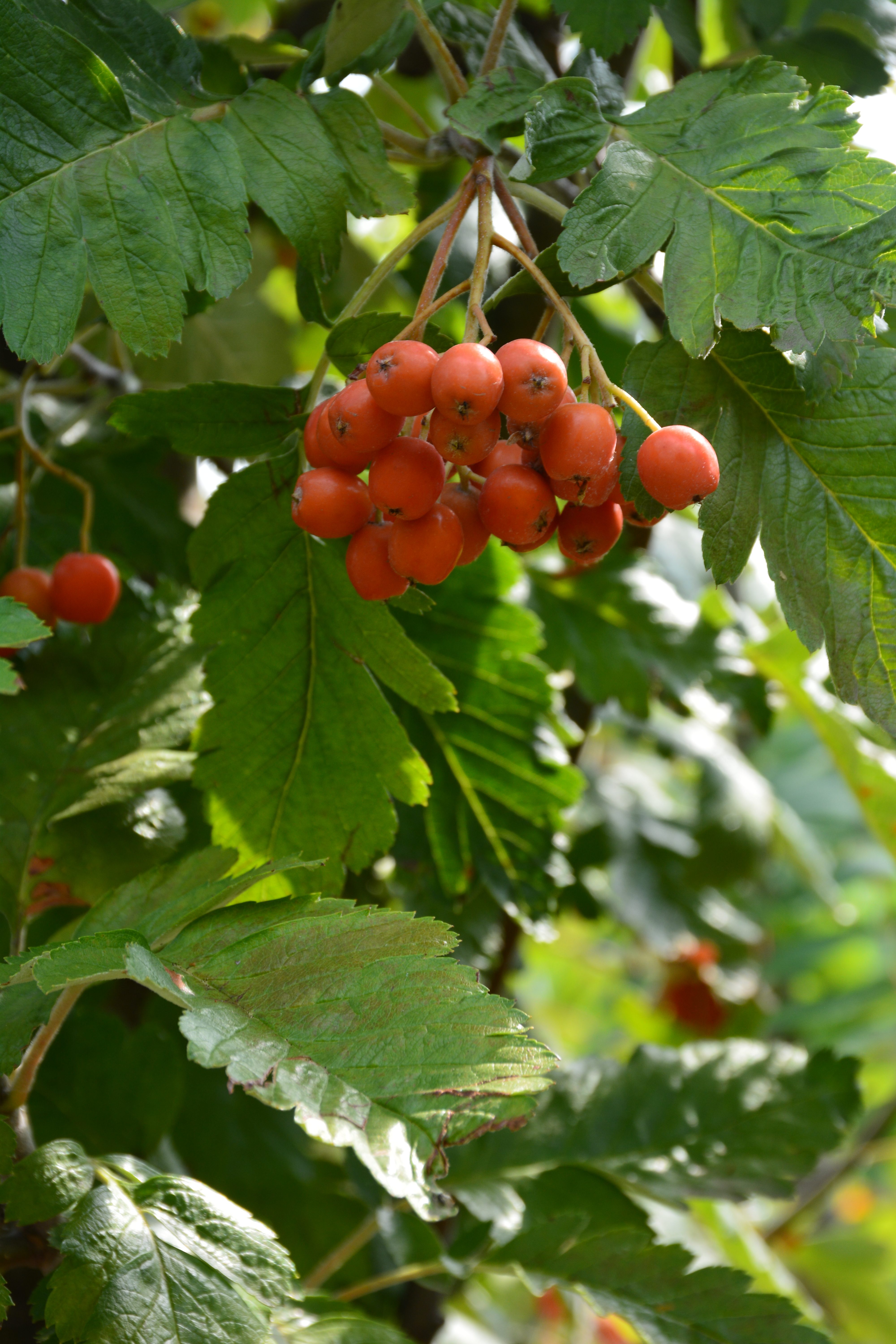This photograph captures a lush tree or bush with abundant, healthy green leaves that span from the bottom to the top of the image. The leaves are large and serrated, and some show signs of insect damage, although the vibrant, red-orange berries remain untouched by pests. These berries grow in clusters of about 10 to 15, with several distinct bunches scattered across the branches. Each berry has a small black nub at the bottom, reminiscent of apple or tomato nubs, adding to their unique appearance. Although these berries superficially resemble familiar fruits like cranberries or small tomatoes, their exact type is not easily identifiable from the image. The weather appears sunny or possibly overcast, casting a gentle light that enhances the vividness of the greenery and the striking color of the berries.